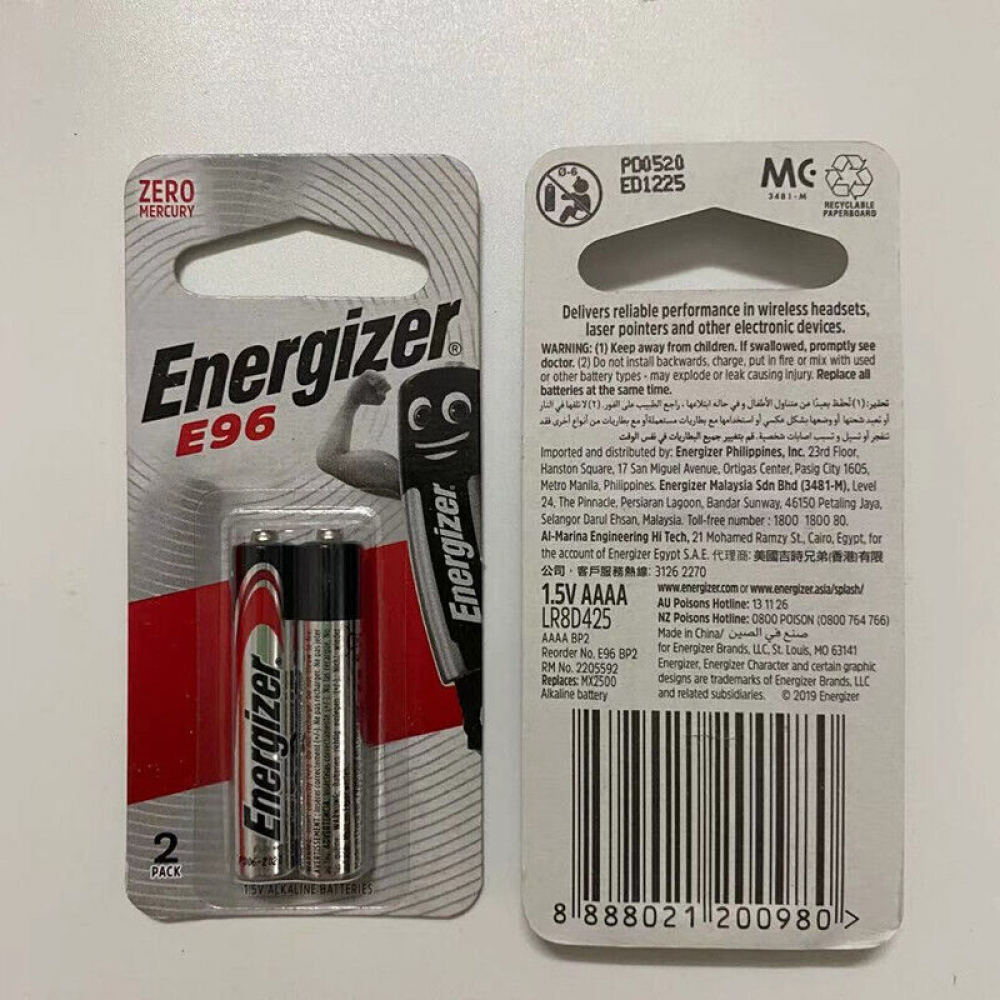The image features a gray background showcasing an Energizer E96 battery pack on the left. The packaging displays two batteries, resembling AA or AAA sizes, prominently marked by a "Zero Mercury" label in the upper left-hand corner. The packaging has a distinctive triangle cutout at the top, designed for hanging on store racks. On the right side of the package, an illustrated black and white Energizer battery character, complete with eyes and a mouth, raises a bent arm to showcase its muscle.

Centered at the bottom, a transparent plastic cover securely houses the two batteries. In the lower left-hand corner, a bold black number "2" stands out, with the word "PACK" emblazoned below it in black against a white background. The package itself is predominantly gray, with a thick red strip running across the bottom.

On the right side of the image, the back of the same package is visible. At the top left, a circle with a diagonal line warns against improper disposal. Various numbers and letters are scattered across this side, accompanied by a recycle icon on the right. Partially obscured text starting with a capital "M" appears to the left. The lower portion of the back features product information and a UPC code at the bottom.